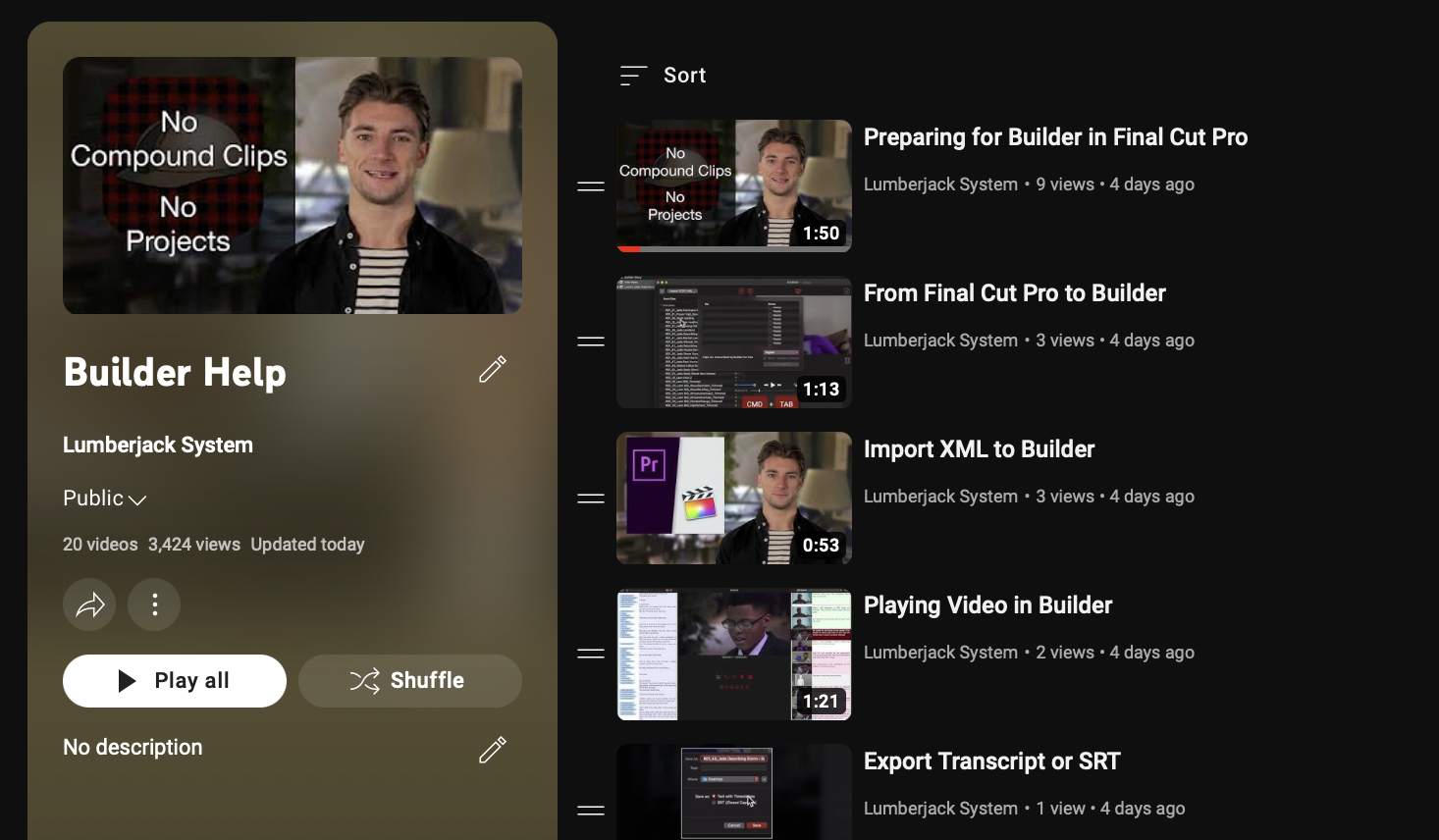The image depicts a dark-themed desktop or tablet screen showcasing a video playback application. The screen is principally black in the background. The application is dedicated to a series named "Builder Help," and it is managed by an account or user called "Lumberjack System." On the left side of the screen, pertinent information about the video collection is displayed: it contains 20 videos, has amassed 3,424 views, and was updated today. There are also buttons for "Play All" and "Shuffle" available for user interaction.

On the right side, a list of available videos is presented, each accompanied by a thumbnail image to their left. The titles of the listed videos are as follows: 

1. "Preparing for Builder in Final Cut Pro" – which appears partially watched, indicated by a red progress bar at the bottom.
2. "From Final Cut Pro to Builder"
3. "Import HML to Builder"
4. "Playing Video with Builder"
5. "Export Transcript or SRT"

Each video title is complemented by a small screenshot, providing a visual snippet of its content.